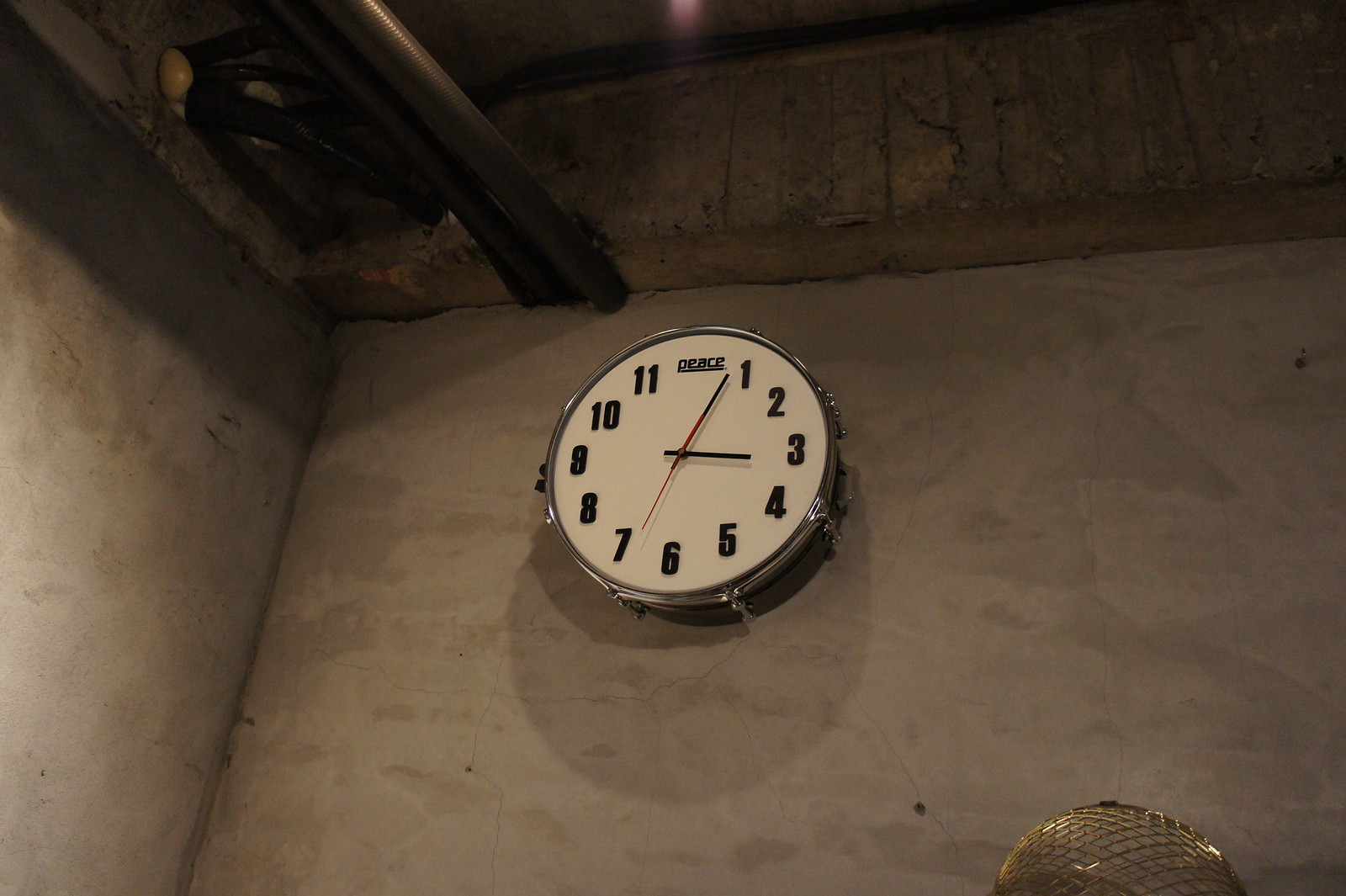The photograph features a wall-mounted clock set against a multi-shaded grey concrete wall. The clock is positioned towards the upper section of the wall, with parts of dark wooden ceiling beams visible above. The lighting in the image is particularly dim and atmospheric, casting pronounced shadows that add depth and a sense of mystery to the scene. 

The clock itself is framed by a sleek silver rim, and the face of the clock is white. Unique to this clock, the space where the number 12 would usually be is replaced by the word "peace" in black lettering. The numerals running from 1 to 11 are bold and italicized, offering an artistic twist. The clock features black hour and minute hands, accompanied by a contrasting red second hand, and it shows the time as slightly past three o'clock. Additionally, a gold metal object occupies the bottom right corner of the image, adding an extra element of intrigue.